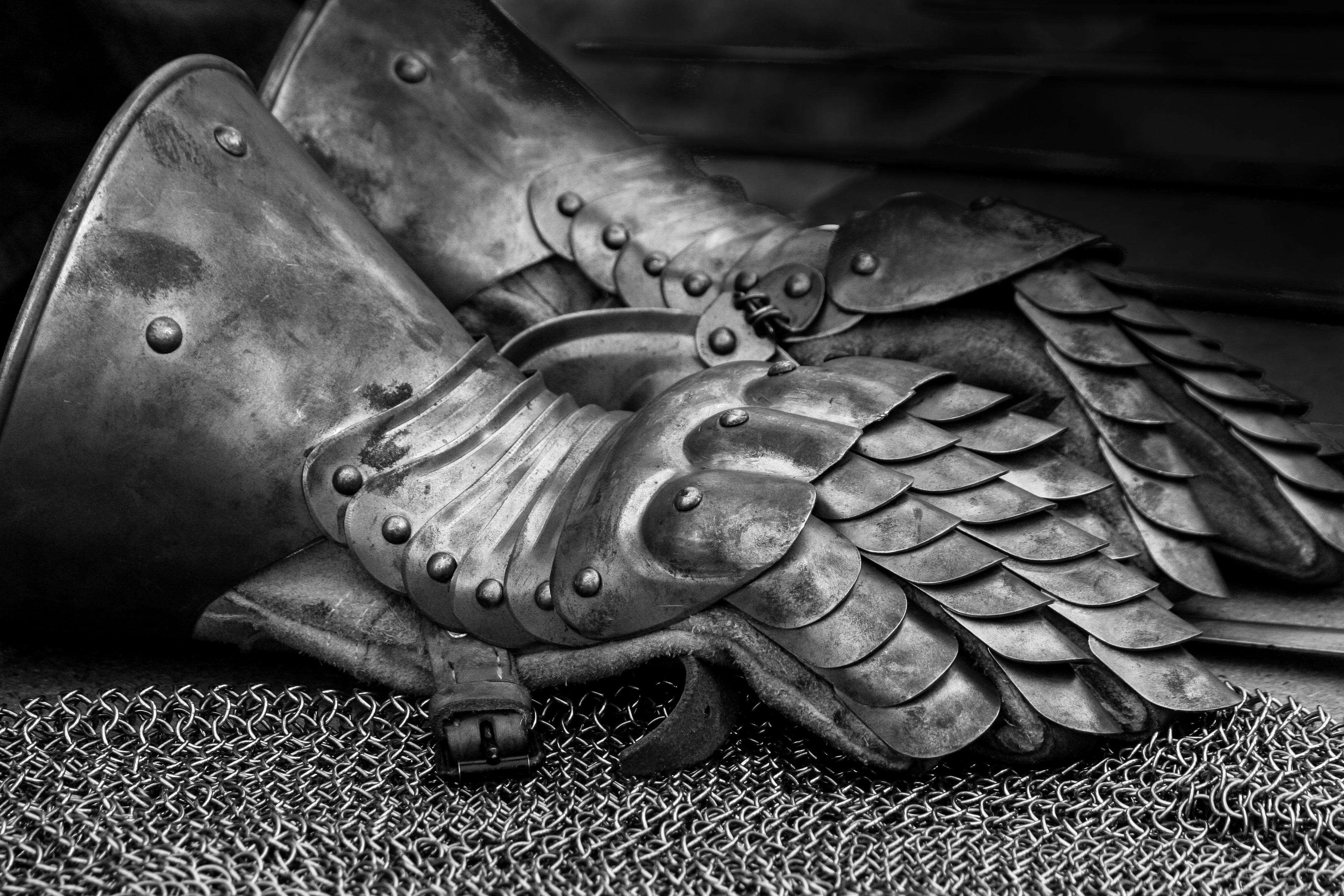This black-and-white photograph captures a detailed close-up of medieval armor with an artistic play of light and shadow. In the foreground, intricate chain mail glistens with a silvery texture, showcasing its elaborate craftsmanship. Resting atop the chain mail are armored gloves designed to resemble scales, extending over the finger area. The gloves display visible rivets and buckles that secure them, alongside subtle fabric outlines. The meticulous quality of the image highlights the texture and detailed construction of the armor. Shadowing towards the corners adds depth and dimension, emphasizing the gloves’ prominence. A touch of dirt is noticeable on the surface of one of the gloves, giving a sense of historical authenticity to the scene. This remarkable image, with its excellent composition and shadowing, evokes a strong sense of artistry and medieval heritage.